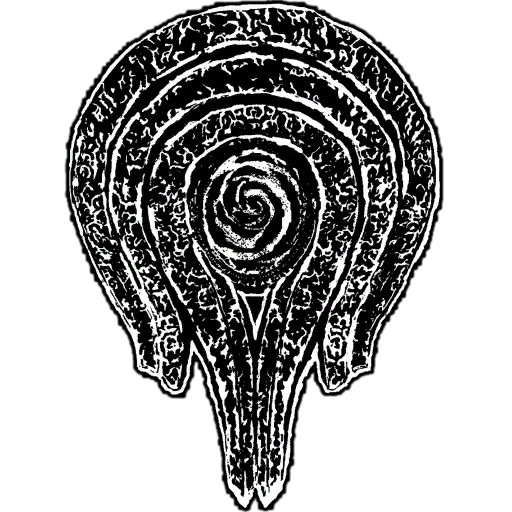The image appears to be a detailed black-and-white drawing or design set against an all-white background. The main form of the image is predominantly round with a notable extension at the bottom, giving it a somewhat snail-like appearance. Central to the image is a spiral, reminiscent of a tightly coiled cinnamon roll, that forms a layered effect. There are around three to four distinct layers, each comprising progressively larger lines. The outermost layer curves into a horseshoe shape, while subsequent layers follow suit but are smaller and intricately close up, creating a pointed effect where the ends meet. Between each of these lines, there is a black, scribbly texture that may represent either shading or a specific pattern. The lower protruding section of the circle is adorned with the same spiral and black scratchy texture. Overall, the design could evoke various interpretations, including sci-fi or even religious symbols, due to its abstract and complex nature.